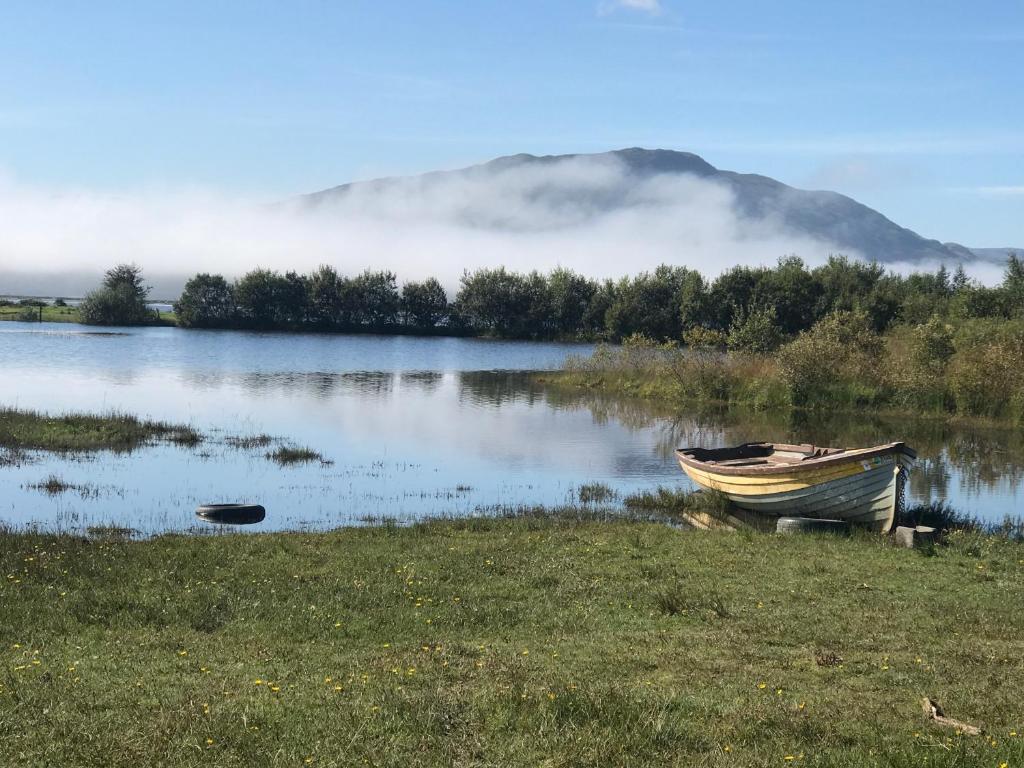This outdoor photograph features a serene and detailed natural landscape. In the foreground, a patch of short, green grass is dotted with small, yellow wildflowers. A weathered rowboat, colored with shades of seafoam green, yellow, and brown, rests partially on the grass and half on the edge of a calm lake. Near the boat, an old tire and some scraps add a touch of rustic abandon. To the left, another tire is half-submerged in the tranquil water, which is bordered by low grass and bushes. The mid-ground is lined with dark green trees standing against the horizon. Layered behind them, dense fog or thick clouds obscure a wide, sprawling mountain, creating a dramatic backdrop. Despite the fog, the sky above is a bright, clear blue, punctuated with only a few wisps of clouds, adding a peaceful ambiance to the scene.